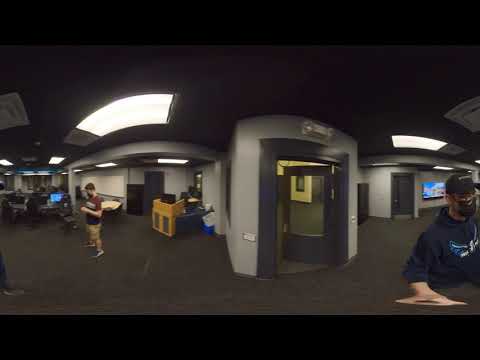In a dimly lit library-like setting, the scene centers around a grey door with a glass insert, positioned in the middle of the space under a black ceiling adorned with white rectangular lights. The floor is dark grey, adding to the room's overall somber tone. To the left of the door stands a man in a brown short-sleeved T-shirt and light brown shorts. Farther back on the left side, a series of long tables with computer monitors are visible, one monitor notably glowing bright blue, and several people are seated at these desks. On the right side of the image, another man wearing a dark blue hoodie with a sports team emblem, a black cap, and a black mask is seated, his hand resting on what appears to be a desk or document. The image itself is framed with a thick black border at the top and bottom, and while some parts appear slightly distorted, the details of the ceiling lights, flooring, and the people present are clear and vivid.